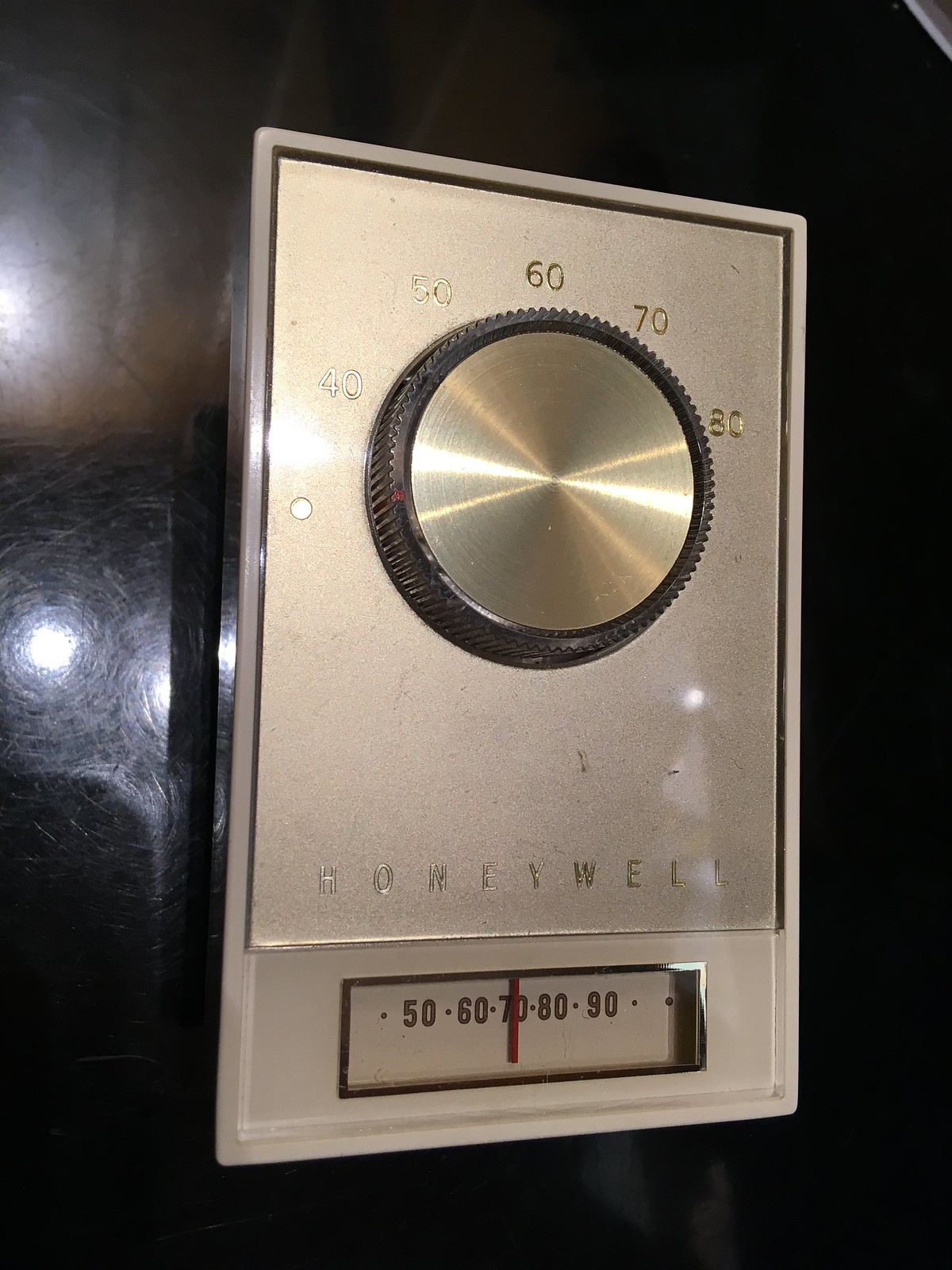This photograph captures a wall-mounted thermostat with a sleek, metallic housing. The housing is rectangular and features a silver finish. Central to the device is a large, tactile knob designed with grooves along its edge for easy grip. The periphery of the knob is black, adding a contrasting border to the brushed metallic circle at its core. Surrounding the knob are engraved gold numbers indicating the temperature settings, ranging from 40 to 80 degrees. Below the knob, the brand name "Honeywell" is prominently displayed in gold text. Beneath this branding, there is a rectangular temperature gauge with a silver border and a red needle indicating the current temperature. The overall design exudes a vintage aesthetic while maintaining functional clarity.